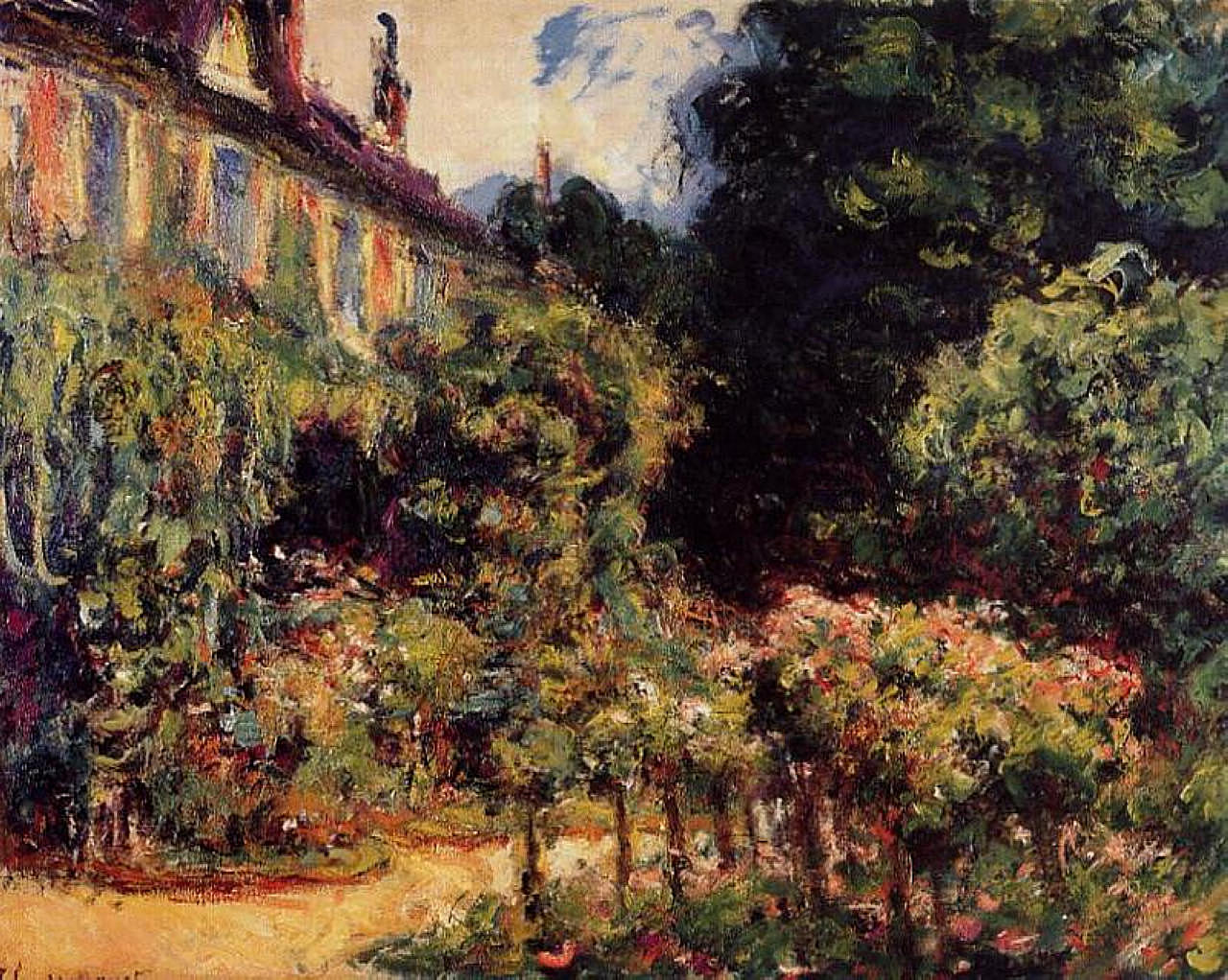This detailed, color painting titled "The Artist's House at Giverny, 1913" by Claude Monet, epitomizes the Impressionism style. The landscape-oriented composition features a vibrant garden path in the foreground, painted in orangish-yellow hues that cut through a lush array of shrubbery and blooming flowers. A large green tree dominates the right side of the image, with meticulous shading that transitions from darker tones at the top toward lighter shades near the front. 

To the upper left portion of the painting stands a picturesque, cottage-like house characterized by its pink and blue paneling mixed with green highlights, and a roof painted in a purplish-plum color. The house features wood-toned shutters, a brown roof with a beige dormer, and a chimney-like structure extending from its right side. The garden blooms vigorously around the house, with additional trees framing the scene.

In the background, a small section of the sky peeks through, painted with swirls of blue and white that are characteristic of Monet's style. The sky is overcast and cloudy, adding a dreamlike quality to the painting. Interestingly, a tower emerges amongst the clouds, adding another layer of depth to the backdrop. Overall, the painting is a rich blend of colors and textures, embodying the essence of Monet's work.